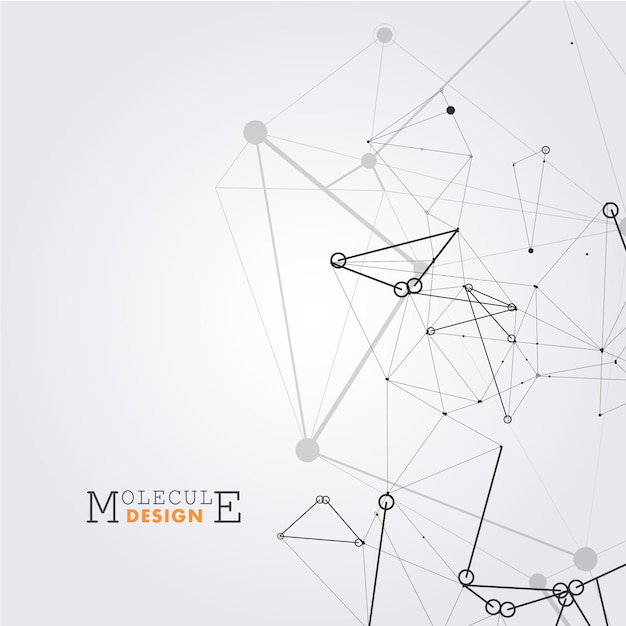This image presents an intricate molecular design, dominated by a mostly off-white background interspersed with black and gray engineering lines and shapes. The design is an abstract yet partially readable structure composed of interconnected polygons, triangles, and circular nodes, some of which are open white circles and others fully closed black ones. These components overlay and interweave to form a complex, visually engaging pattern. The bottom left corner of the image features the logo "Molecule Design", with a large capital "M" and "E" on either side of the word "Design" written in a bold font, colored in orange. The entire composition gives off a technical, engineered feel with its meticulous arrangement of lines and nodes.